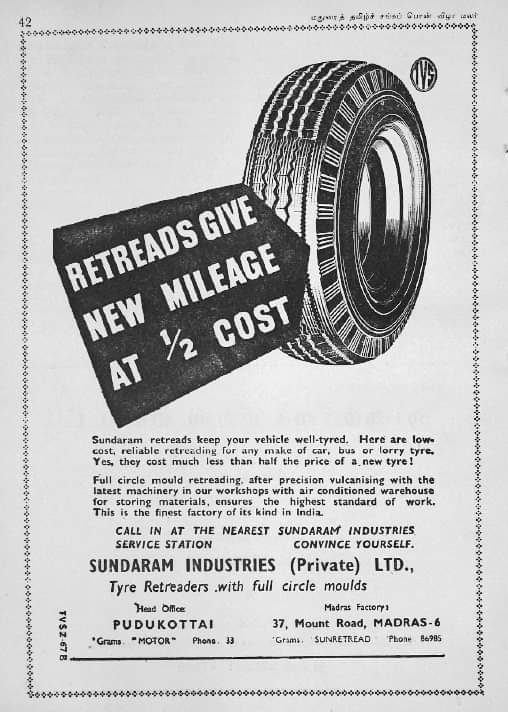This detailed black-and-white advertisement from a vintage publication is for Sundaram Industries, a renowned tire company in India. The ad, found on page 42 and bordered by a pattern of small black diamonds forming a rectangle, promotes their cost-effective retread tires. Dominating the top right of the ad is a large tire image, with its tread structure prominently displayed. To the left, a black trapezoid with white text declares, "Retreads give new mileage at half cost." Below this bold statement, two paragraphs explain the benefits of Sundaram's retread tires, emphasizing their affordability—costing much less than half the price of new tires—and their reliability for any make of car, bus, or lorry. The ad mentions Sundaram’s cutting-edge retreading process, utilizing full-circle mold retreading and precision vulcanizing with the latest machinery, all conducted in their air-conditioned warehouse to ensure top-notch quality. The company is highlighted as having the finest factory of its kind in India. At the bottom of the ad, the name Sundaram Industries (Private LTD) is displayed, along with contact information for two locations: Pudukottai and Madras. For further details, readers are encouraged to visit the nearest Sundaram industry service station.